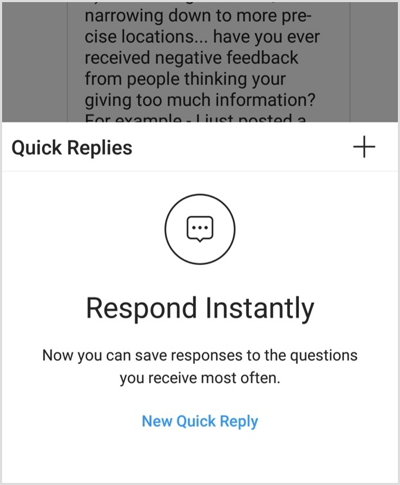The image appears to be a screenshot from a mobile device, likely an iPad, featuring the Instagram Direct Messages (DMs) interface. The central focus is on the "Quick Replies" feature, which allows users to save responses to frequently asked questions for faster replies. In the upper right section of the screenshot, there is a plus button, which users can tap to add new quick replies. The screenshot includes instructional text that reads, "Quick replies: respond instantly," and "Now you can save responses to the questions you receive most often."

In the background, partially obscured by the quick reply overlay, is a snippet of a direct message, where the visible text reads: "narrowing down to more precise locations. Have you ever received negative feedback from people thinking you're giving too much information? For example, I just posted...". The remaining portion of the message is hidden beneath the overlay. Given the context, the image seems to be demonstrating how the quick replies feature can be used, likely intended for individuals with large followings, such as celebrities or influencers, to efficiently manage their interactions on Instagram.